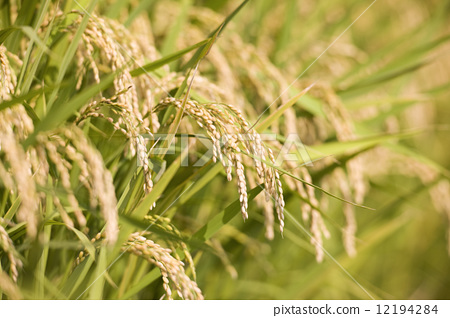This professionally shot, outdoor image, likely captured during daytime due to its brightness, is a stock photo available on Pix2Stock.com, with a visible watermark reading 'Pixta' and the number '1219-4284'. The photo vividly depicts a close-up view of a field of grain, possibly wheat, amidst tall green leaves. The central focus is on the tall stems bearing tan kernels, characteristic of wheat or oats, which appear slightly drooping and are reminiscent of ribbons. The image features a narrow depth of field, with only a portion of the grain in sharp focus while the background and edges blur, emphasizing the detailed texture and natural growth pattern of the grain.